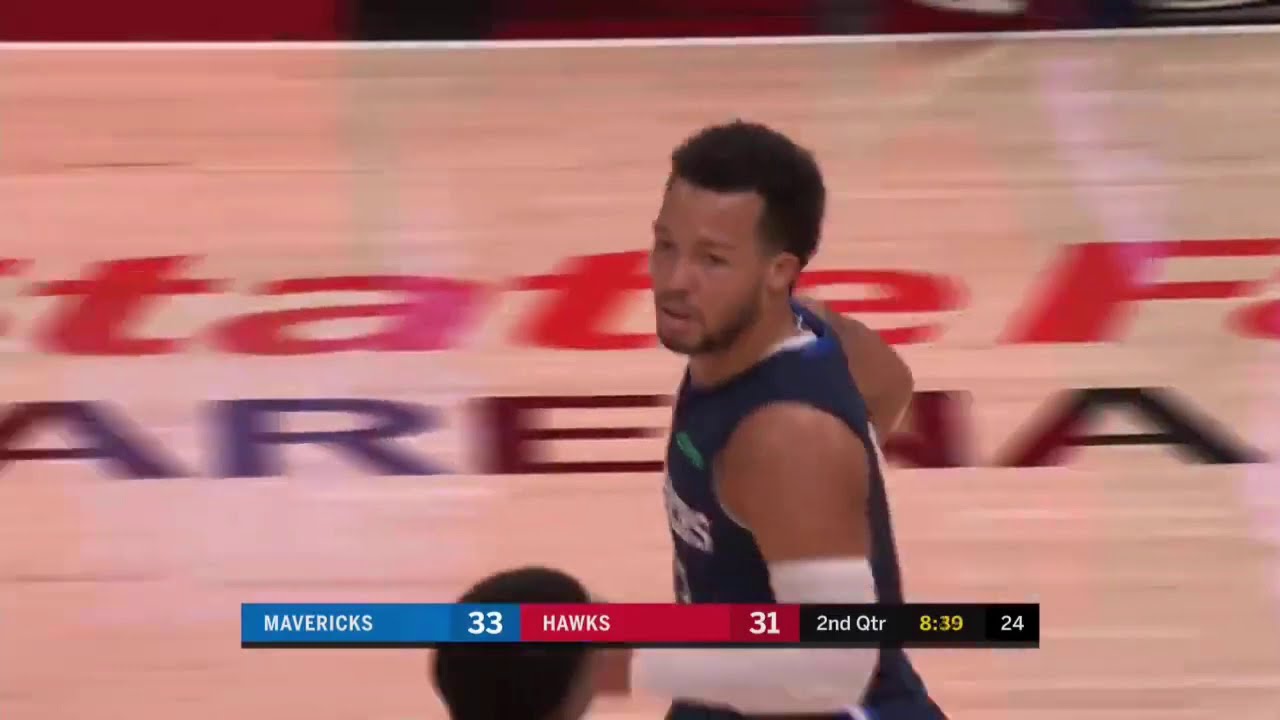The image is a still photograph taken from a TV broadcast of an NBA basketball game between the Dallas Mavericks and the Atlanta Hawks, set in State Farm Arena, Atlanta. It captures Jalen Brunson, a light-skinned black player with short black curly hair and a trimmed beard, running down the court. He is seen from the waist up, wearing a dark blue Mavericks jersey with white text, and a white shooting sleeve extending from his bicep down to his wrist. The score displayed at the bottom of the image shows the Mavericks leading with 33 points to the Hawks' 31, indicating it's the 2nd quarter with 8 minutes and 39 seconds left on the game clock and 24 seconds on the shot clock. The captured motion causes a slight blur on the court, emphasizing the in-game action. The State Farm Arena markings are partially visible on the hardwood floor. Another player's head with curly black hair is seen at the very bottom of the image.